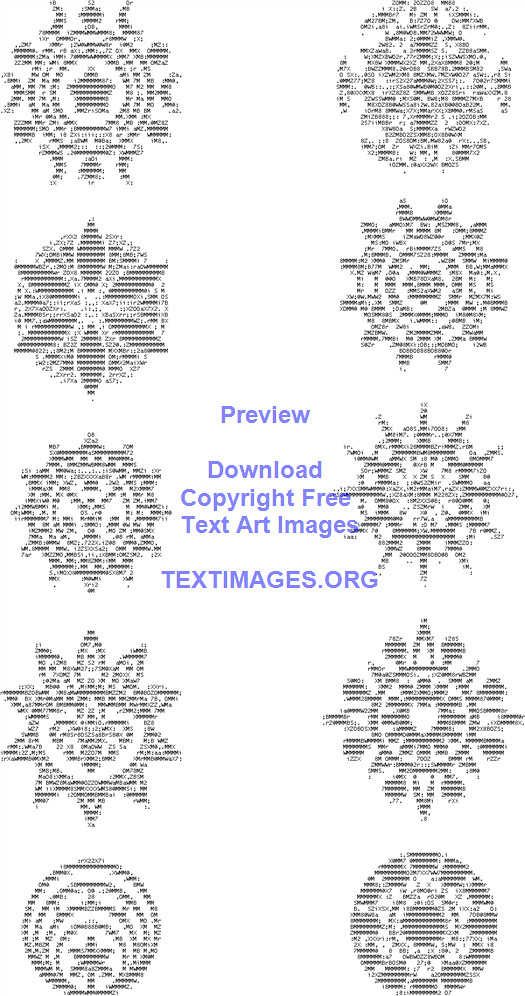The image is a digitally synthesized artwork featuring 10 symmetrical symbols arranged in two vertical columns of five on either side, against a white background. Each unique symbol appears to be composed of small, black-colored characters—possibly numbers, letters, or other symbols—creating a textured, grayish appearance. These intricate symbols resemble snowflakes or flowers with rounded, star-like shapes. In the center, in blue text, the image prominently displays the words "PREVIEW, DOWNLOAD, COPYRIGHT FREE, TEXT ART IMAGES, TEXTIMAGES.ORG." followed by "TEXTIMAGES.ORG" in all capitals. The overall composition blends the precise symmetry of the symbols with the informative blue text, creating a visually engaging piece.